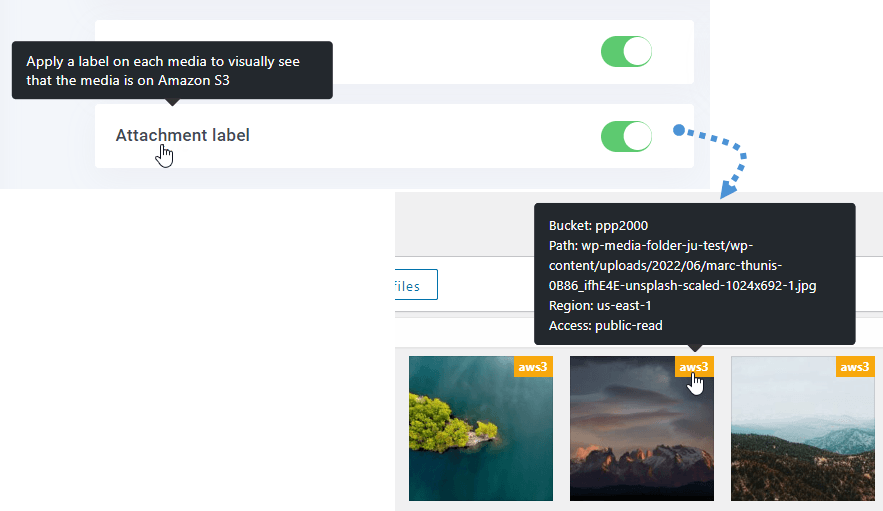The image consists of two distinct screenshots that have been spliced together. In the first screenshot, there is a partial view of what appears to be an iPhone interface, showcasing two toggle buttons similar to the iOS design where a gray circle signifies 'off' and green signifies 'on.' The first toggle button is obstructed by a black information box, making its label unreadable. The second toggle is labeled "Attachment Label," and hovering over it triggers a black tooltip that states, "Apply a label on each media to visually see that the media is on Amazon S3."

In the second screenshot, there are three thumbnail images arrayed in tiles, each depicting different landscapes. One image shows an island, another captures a mountain range at dusk, and the third represents a different mountain range. A cursor is hovering over the second image, causing a black information box to appear. The tooltip provides detailed metadata about the image, listing the path as "bucket PPP 2000 > path WP > me > folder your JU > test / WP > content-uploads-2022-06 mark-soonest-OB86-IFHE4e-unsplash-scaled-1024x692-1.jpg," and further information specifies the region as "US East 1" and the access level as "public."

This descriptive caption encapsulates the intricacies observed in the screenshots, illustrating the UI elements, image details, and technical metadata presented.